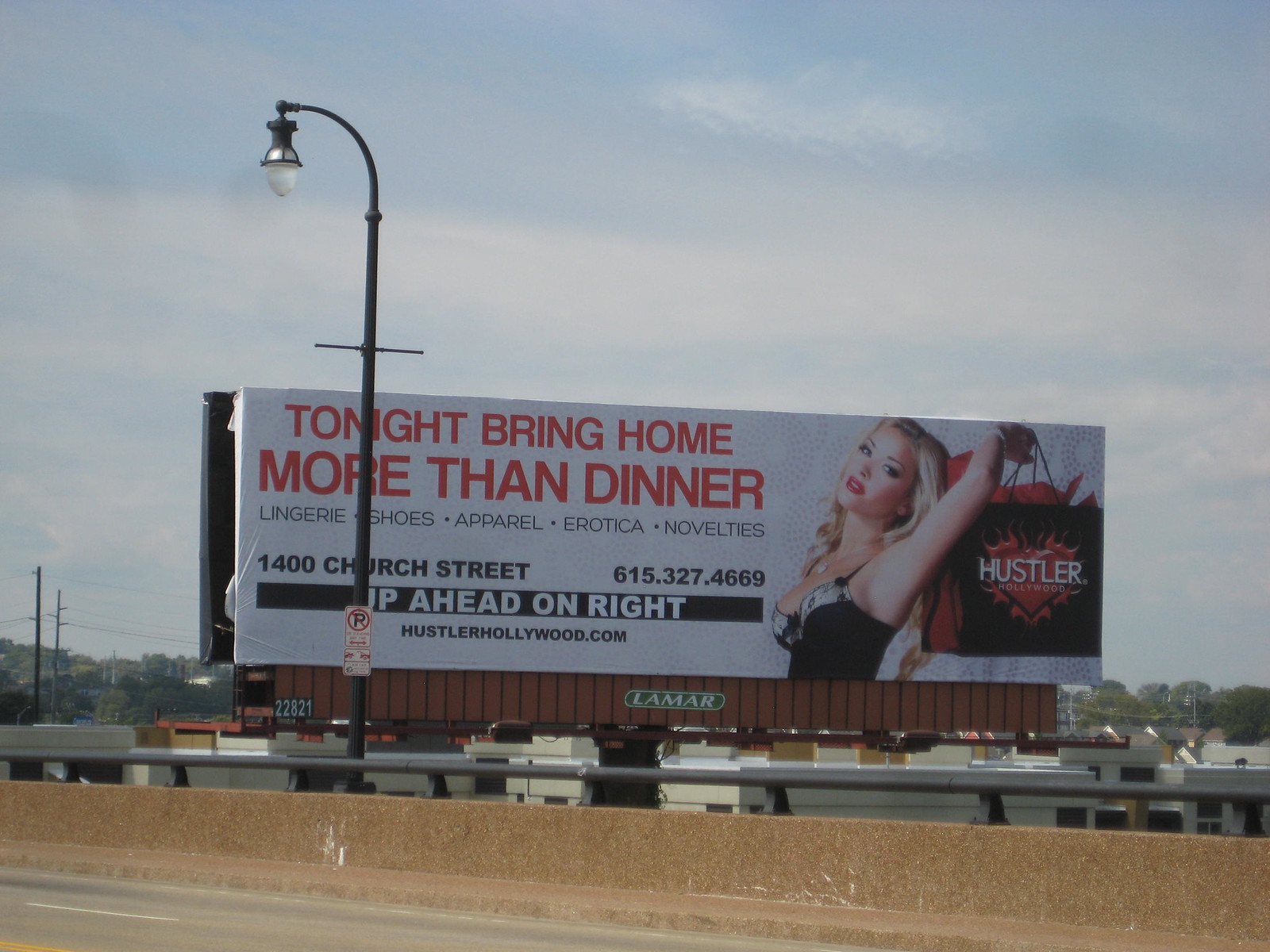This photograph captures a bustling highway scene with a prominent billboard as the focal point. In the foreground, there's a stretch of highway flanked by a sturdy concrete barrier, which is topped by a familiar metal guard rail for added safety. The viewer's eye follows the scene to the middle left where a lone street light punctuates the landscape, adding an urban touch to the setting. Beyond the barrier, glimpses of buildings can be seen, suggesting a backdrop of a cityscape.

Dominating the scene is a large billboard featuring a striking image of a woman in an alluring pose, holding a Hustler bag. Bold text on the billboard reads: "Tonight, bring home more than dinner," followed by a list of available items including lingerie, shoes, apparel, erotica, and novelties. The billboard also provides specific directions, stating "1400 Church Street, up ahead on the right," alongside a website and phone number for more information. This billboard serves as an advertisement for Hustler, adding a touch of provocative allure to the everyday highway environment.